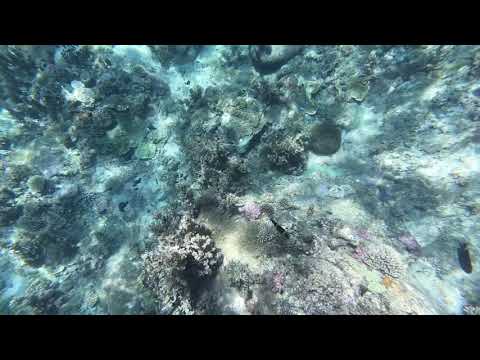This is a detailed top-down aerial shot of a brightly lit coral reef underwater. The image showcases a vibrant array of colors ranging from dark bluish-green, through lighter brownish hues, to purple lavender and even yellow tones towards the front. Amidst the coral, there are several sea creatures including possible anemones, a starfish, and a few fish. Notably, there's a black fish near the right side and the shadows of other fish shapes in the bottom right corner. The setting appears to depict the bottom of the ocean with mixed elements like rocks, seaweed, and waves, adding to the dynamic nature of the scene. The entire picturesque view is framed with a six-inch black border at the top and bottom, encapsulating the diverse aquatic landscape.